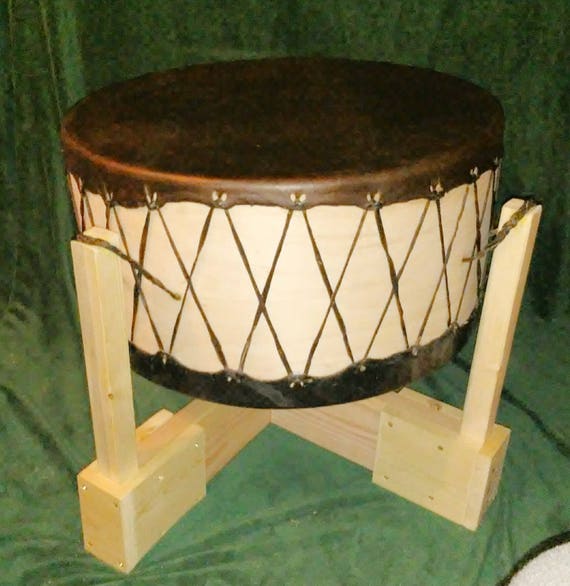A detailed indoor color photograph of a lightly used drum made of natural, light tan wood. The drum features a tightly strung dark brown animal skin membrane secured in a distinctive crisscross pattern around its circumference with matching brown ropes. It is neatly placed in an X-shaped wooden stand, likely made from maple, with visible gold or silver screws marking the joints. The drum and its stand are positioned against a green cloth backdrop that drapes from the floor up behind the drum. Additionally, there are small rope handles attached to the drum for easy carrying. The overall scene suggests that the drum is more for display than for active use.